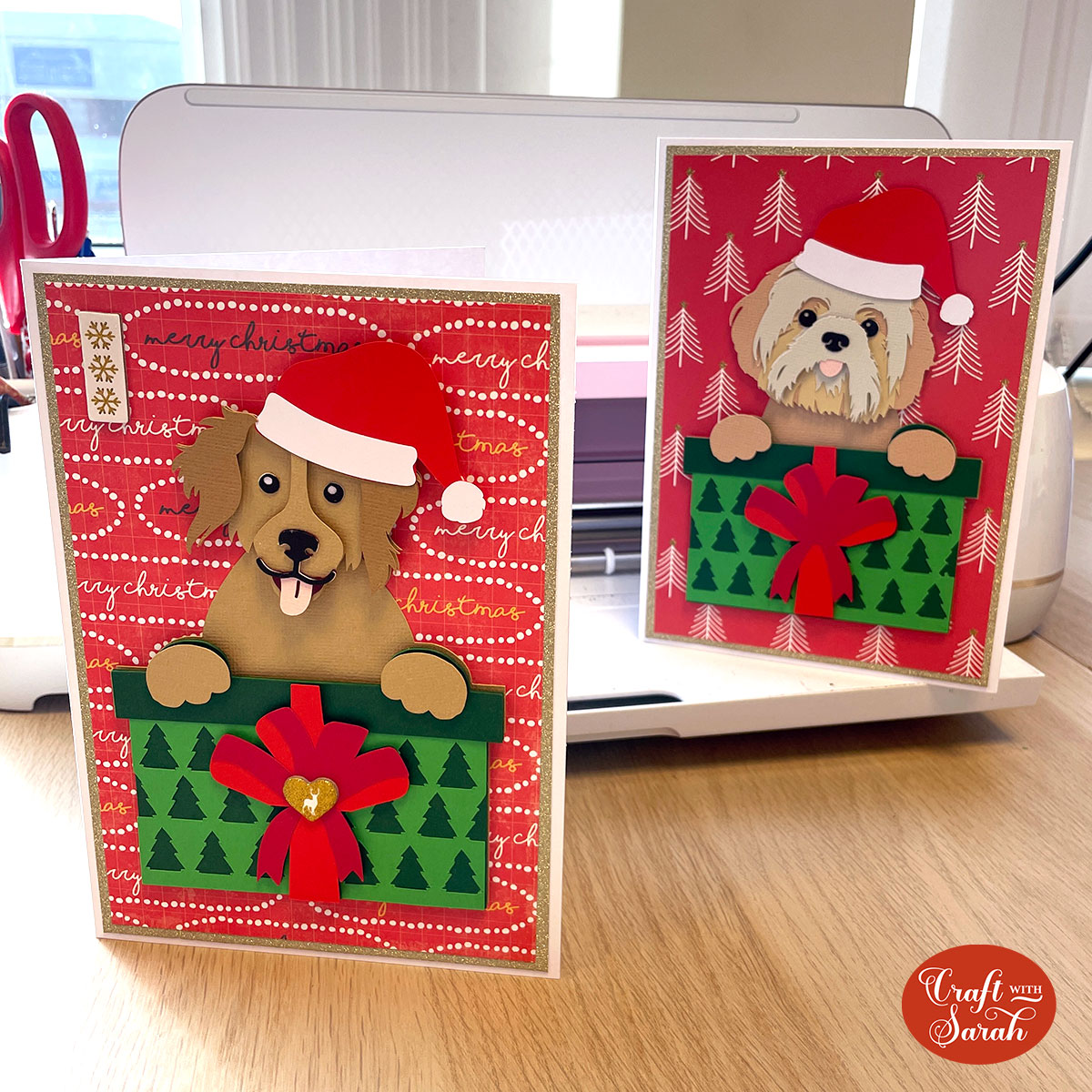This detailed photograph showcases a creative setup featuring two 3D Christmas greeting cards prominently placed around a white Cricut machine on a wooden desk with a window and blinds in the background. The machine, known for cutting stencils and vinyls, holds red scissors in its storage pocket, contributing to the crafting theme. Both cards share a similar aesthetic with a festive red background and dual borders, one white and one gold. The card on top of the machine displays a fluffy tan puppy in a Christmas hat, perched on a green present with a red bow, set against a backdrop of white-drawn Christmas trees. The puppy lovingly gazes outward with its tongue sticking out. 

The second card, positioned in front of the machine, mirrors the festive look but with distinctive elements. This card also features a tan fluffy puppy, likely a Shih Tzu, adorned with a Santa hat and similarly playful expression, resting its paws on a Christmas box. This pup is seen amongst colorful dots surrounding the greeting "Merry Christmas." Additional details like a white cup, pins, and red scissors scattered in the background breathe life into the crafting scene, suggesting a bustling workspace where these charming cards are thoughtfully created.